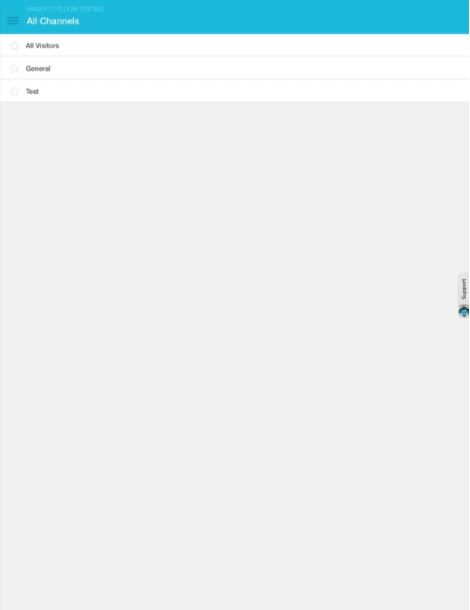This image appears to be a screenshot taken from either a computer or a mobile device. At the very top, there is a teal-colored header with the text "All Channels" in white located in the upper left corner. Below this header, the screen is divided into three vertical sections on the left side. The sections are labeled from top to bottom as "All Visitors," "General," and "Test," each separated by a light gray line.

Beneath the "Test" section, the remaining part of the image consists of a large light gray square. Situated in the top right corner of this gray square is a small rectangular box containing text that is too tiny to discern. Accompanying this box is a blue circular icon to its left. The remainder of the gray area is devoid of any additional text or images.